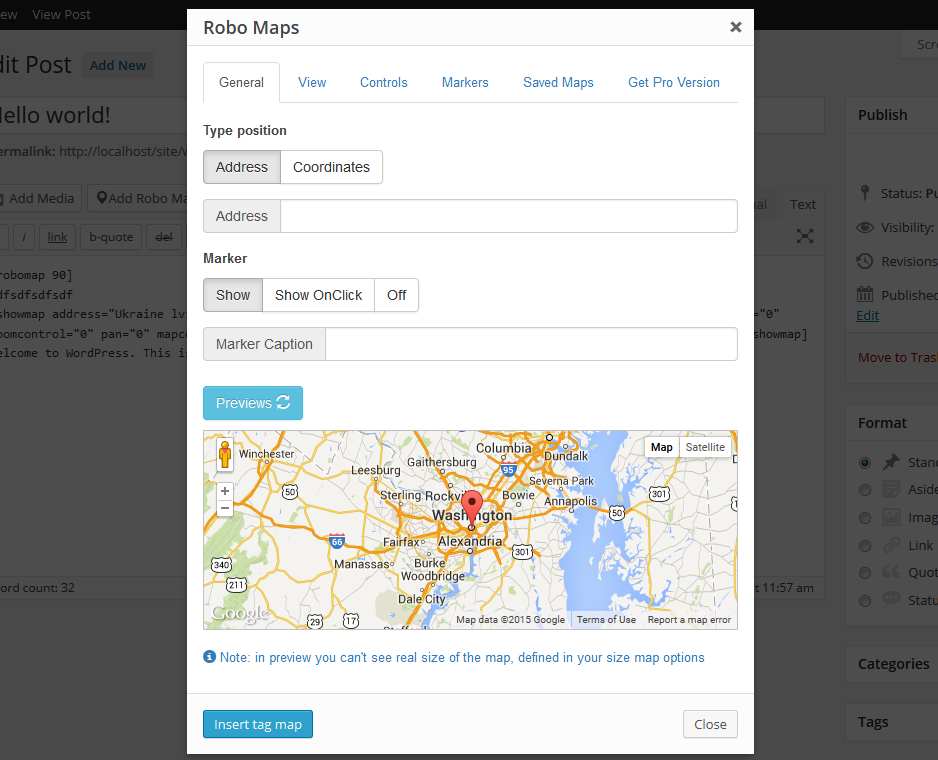**Descriptive Caption:**

The screenshot showcases a section of a user interface for an application named "RoboMaps." At the top, there is a header with the label "RoboMaps." On the top-right corner, there's an "X" icon, typically used to close the window or dialog box. Beneath the header, there's a list of menu options including "General," "View Controls," "Markers," "Save Maps," and "Get Pro Version."

Further down, under a heading labeled "Typo Position," there are two buttons: one is gray with the label "Address," and the other is white labeled "Coordinates." Adjacent to these buttons is a text box for typing in an address.

Below this section, there is another labeled "Marker." Within this section, there's a gray button labeled "Show," a white button labeled "Show on Click," and another white button labeled "Off." Following this, there is a gray button titled "Marker Caption" next to a text box for inputting a caption.

A prominent blue button labeled "Previews" is situated below this array of options. Directly below the "Previews" button is a screenshot of a Google Maps interface depicting a map of Washington, D.C., and its surrounding area, marked with a red location pin.

At the bottom of the screenshot, there's a cautionary note stating, "Note and Preview: You can't see the real size of the map, define in your side map options."